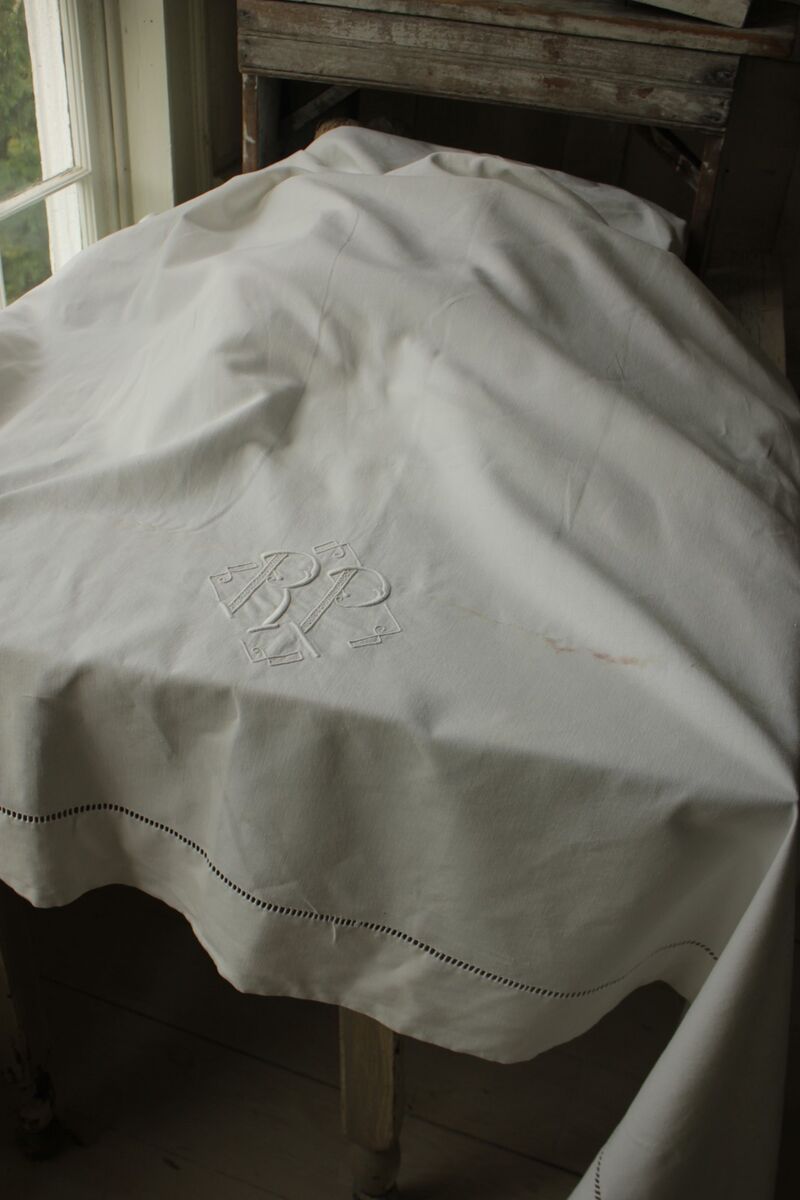This is an indoor photograph of a large white linen cloth, likely a tablecloth, draped over a well-worn, vintage wooden table. The photograph appears aged and of low quality, hinting at its age. To the left, a sash window sheds light on the scene, offering a glimpse of grass outside. The cloth features intricate details, including a series of small perforations near the bottom edge, forming a dashed or dotted pattern. Additionally, the cloth is adorned with a regal-looking monogram that reads "RP," which appears to be sewn in with a sewing machine. The monogram is surrounded by a decorative square, adding to its personalized feel. Behind the table and cloth, there's another piece of old furniture, possibly a cabinet or a mantelpiece, contributing to the vintage ambiance of the setting.